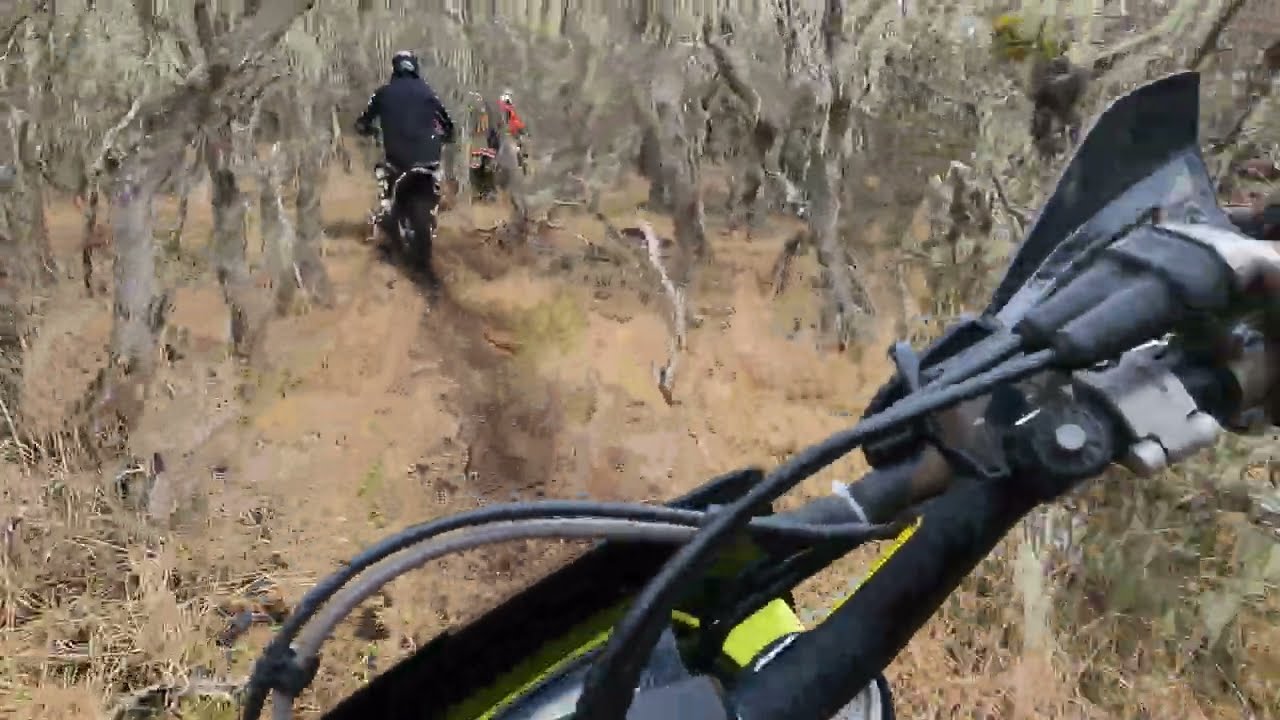The photograph captures the perspective of a rider on a dirt bike, with a focus on the right handlebar, adorned in black with fluorescent yellow accents and a tangle of black wires. The backdrop reveals a rugged trail bordered by half-dead, greyish-brown trees and thick underbrush. The scene is set on a narrow dirt pathway, speckled with darker patches of mud, leading through a dense, somewhat blurry forest. Directly ahead, a fellow biker dressed in a black jacket and helmet dominates the view, with another biker in red and a white helmet faintly visible further along the trail, partially obscured by foliage. The entire atmosphere is one of rugged adventure through a challenging, wooded terrain.